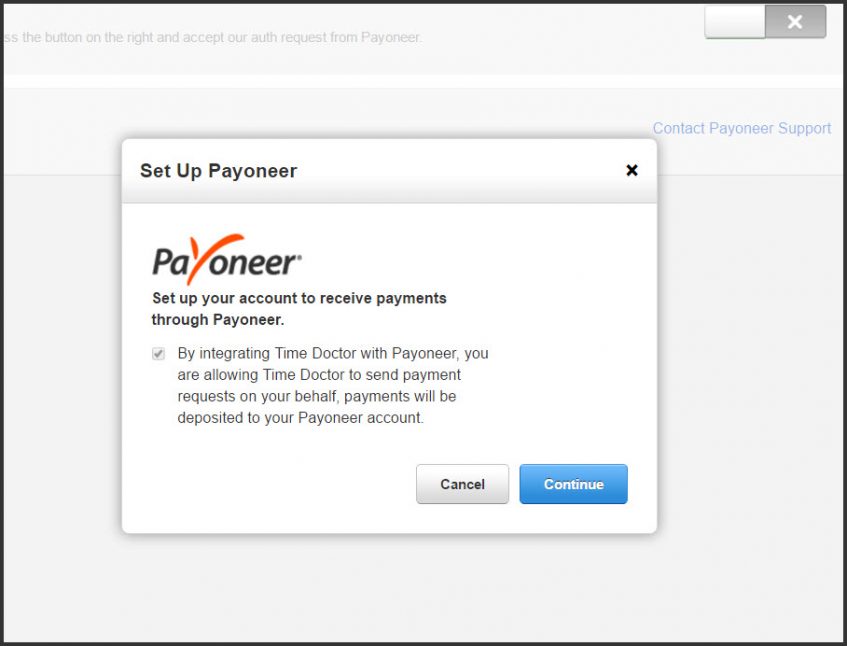This vertical image showcases a webpage accessible via computer or smart device. Framed by a thick black border, the page background features a medium gray tone. 

At the top left corner, partially cut-off text appears to spell "Press" followed by "Accept our auth request from Payoneer." On the upper right, there are two small rectangular boxes: one white and the other gray with a white "X" inside, likely for closing the overlay. 

A narrow white strip runs horizontally beneath these elements, reverting back to the gray background. Just above this strip, positioned on the top right, a blue phrase reads "Contact Payoneer Support."

An overlay box is central in the image, starting with a gray header bar labeled "Set up Payoneer" alongside a black "X" to close it. Below this, a larger white box displays the Payoneer logo and text guiding account setup for receiving payments through Payoneer. It explains that by integrating Time Doctor with Payoneer, users authorize Time Doctor to send payment requests on their behalf, which will be deposited into their Payoneer account.

At the bottom of this white box, options to "Cancel" or "Continue" are presented, with the "Continue" button highlighted in blue.